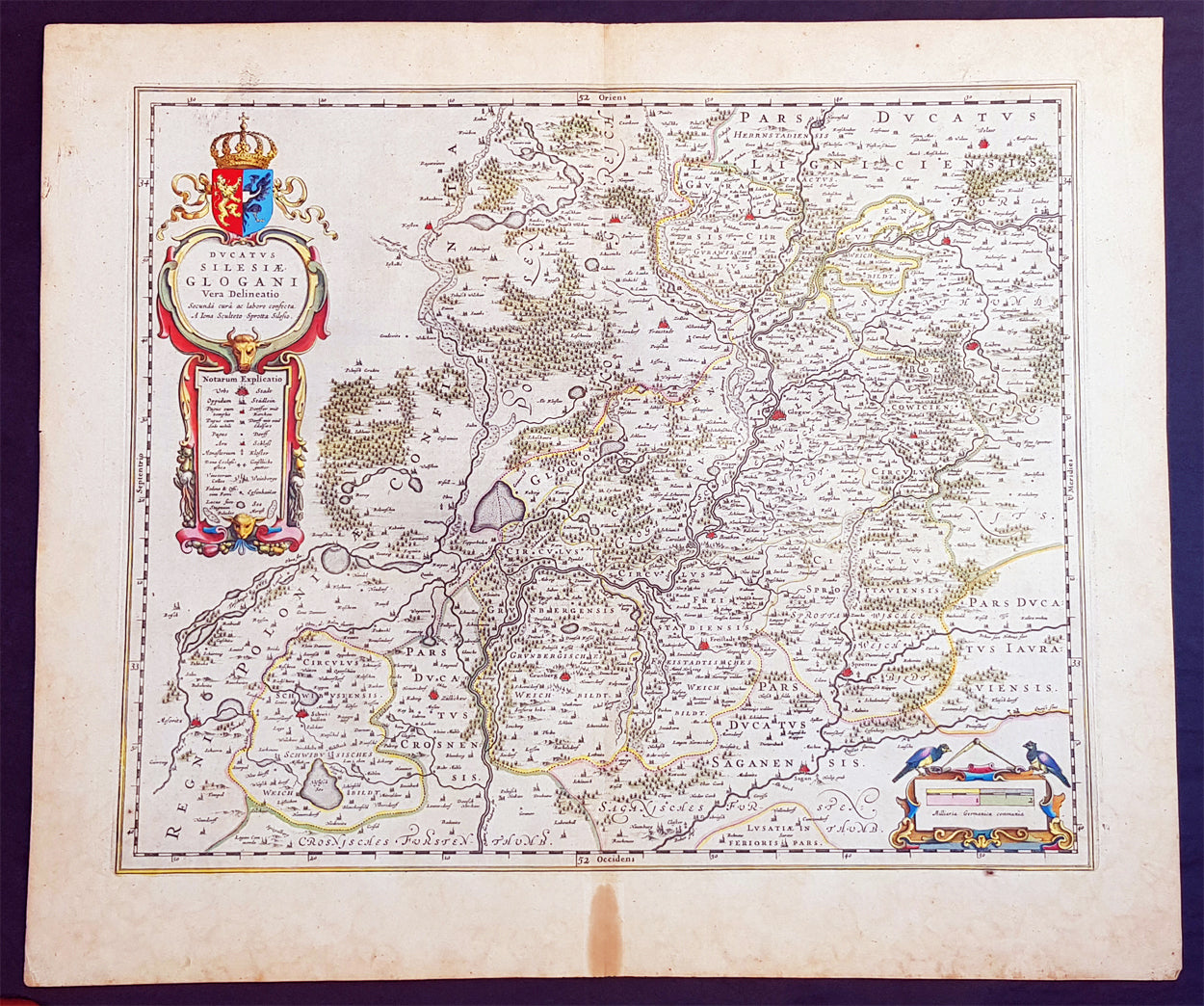This is a highly detailed, framed map that appears to be quite old, suggested by its discolored, mottled paper and Latin text. The map seems to be an early depiction of Europe, possibly featuring the landmasses of Spain and Portugal, although this is not entirely certain. The map is filled with intricate illustrations of various rivers and landmarks, and numerous place names, none of which are in English and thus hard to interpret. Notably, the top right of the map contains the Latin text "PARS DVCATVS."

The map is adorned with several heraldic symbols: on the left side, there is a coat of arms featuring a gold crown with red and blue emblems, while the bottom right showcases a crest with two blue birds. Additionally, a scale is present in the lower right corner, presumably for measuring distances within the map. The overall color scheme includes shades of red, blue, white, and gray. The map’s complex and dense text, along with its congested depiction of numerous small cities, lends it an intriguing and historical aura.